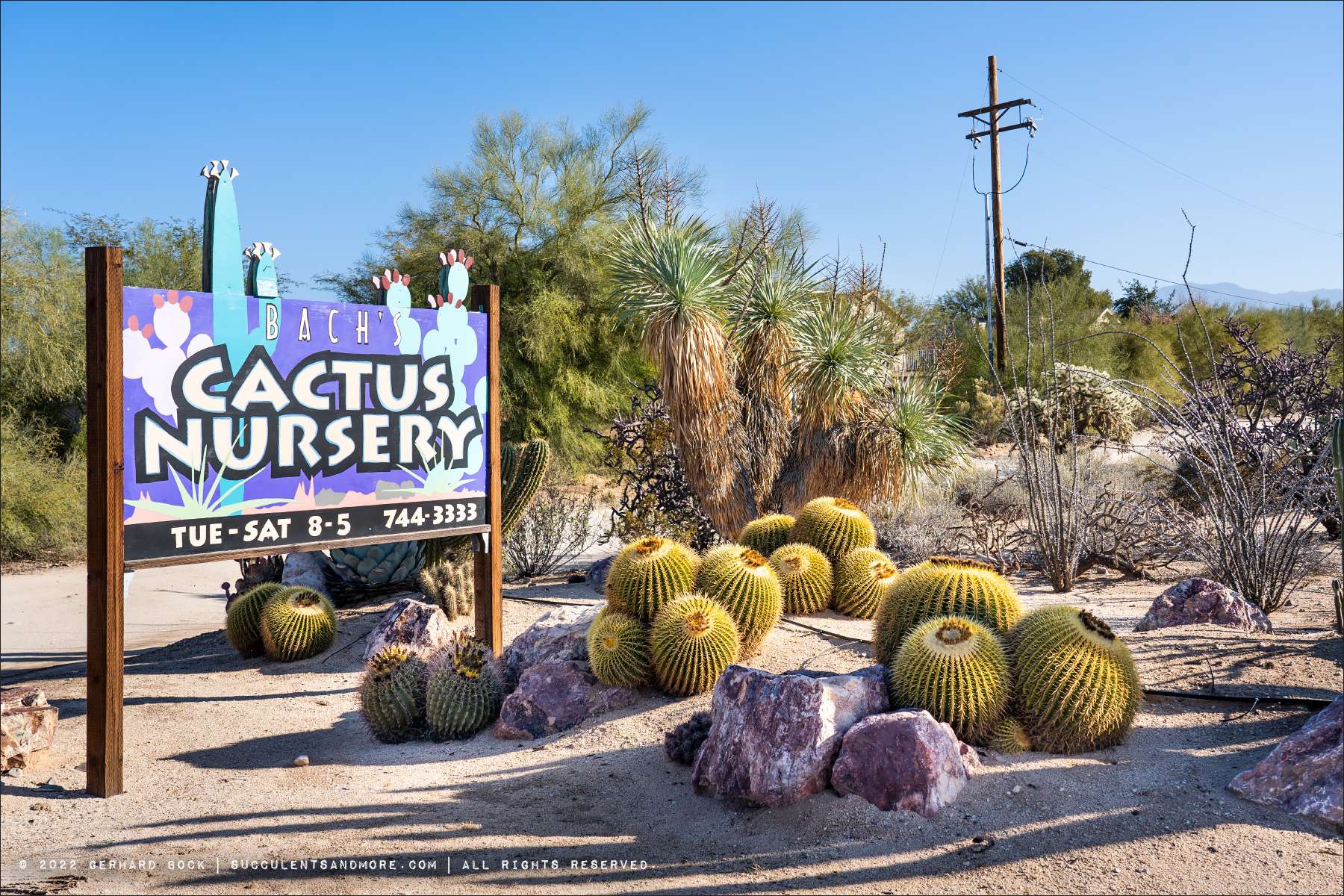This photo captures a vibrant desert scene at Box Cactus Nursery. Prominently on the left side stands a sign with wooden posts, boldly stating "Cactus Nursery" outlined in thick black lettering, with the smaller text "Box" above it. Beneath it lists the hours "Tuesday through Saturday, 8 to 5" and a contact number, "744-3333." The sign is set against a backdrop featuring cutout images of cacti, painted in purples, blues, black, and white, extending beyond the sign's top edge. The supplementary text reads "2022 Gerhard Bach Succulents and More - All Rights Reserved."

In the foreground, clusters of round cacti dot the sandy ground, interspersed with boulders and rocks. Drought-resistant greenery and various desert plants add to the arid ambiance. A tall telephone pole stretches wires to the right, framed by a clear blue sky. The morning light accentuates the textures and colors of the scene, from the spiky cacti that have finished blooming to the distinctive yellow and green stranny desert shrubs. The entire composition beautifully captures the rugged yet thriving desert environment.